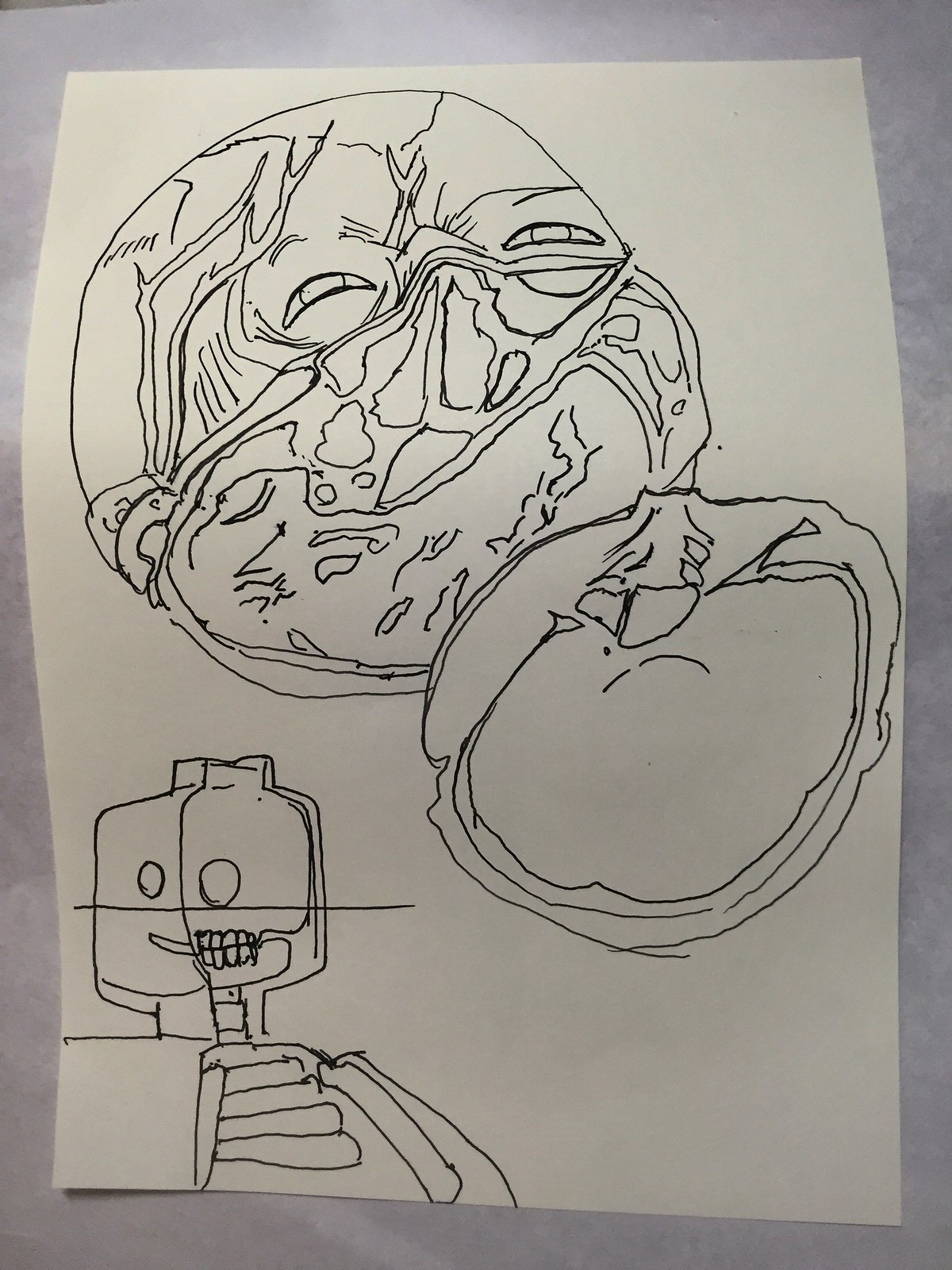The image is a pen drawing on a lightly greyish-white paper, set against a plain light grey background. The drawing features intricate, science fiction-inspired elements that are somewhat abstract and not immediately recognizable. At the bottom of the image, there are steps leading up to a square-shaped face, which displays noticeable eyes and a partially open mouth revealing teeth, though the features are not realistic. Dominating the upper part of the drawing are two large circles filled with various shapes and lines. At the top of the circles, there is an abstract depiction of a human face-like form, with distinguishable eyes. The intricate patterns and shapes within the circles potentially hint at brain-like structures, blending elements of human anatomy with abstract, sci-fi motifs.